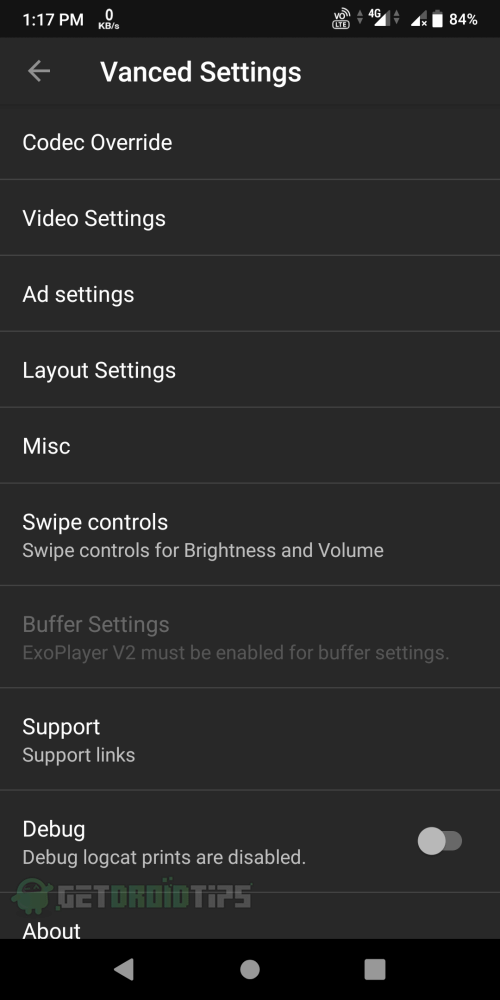This is a detailed caption for an image showing the settings page of a mobile app captured in a screenshot. The screenshot displays a phone interface with the top menu bar indicating battery level, signal strength, and current time, while the bottom menu bar includes the back button, home button, and close all button. The main content shows the advanced settings of the app, titled "Vanced Settings." 

Within these settings, users can find a variety of options including:
- **Codec Override**
- **Video Settings**
- **Ad Settings**
- **Layout Settings**
- **Miscellaneous**
- **Swipe Control**: Includes a description stating that swipe controls manage brightness and volume.
- **Support**: Includes a description stating support links.
- **Debug**: Includes a description stating debug logcat prints are disabled.
- **About**
- **Buffer Settings**: Grayed out with a note indicating that enabling ExoPlayer version 2 is necessary for buffer settings.

The overall interface is set to a dark mode theme, featuring a dark gray or black color scheme.